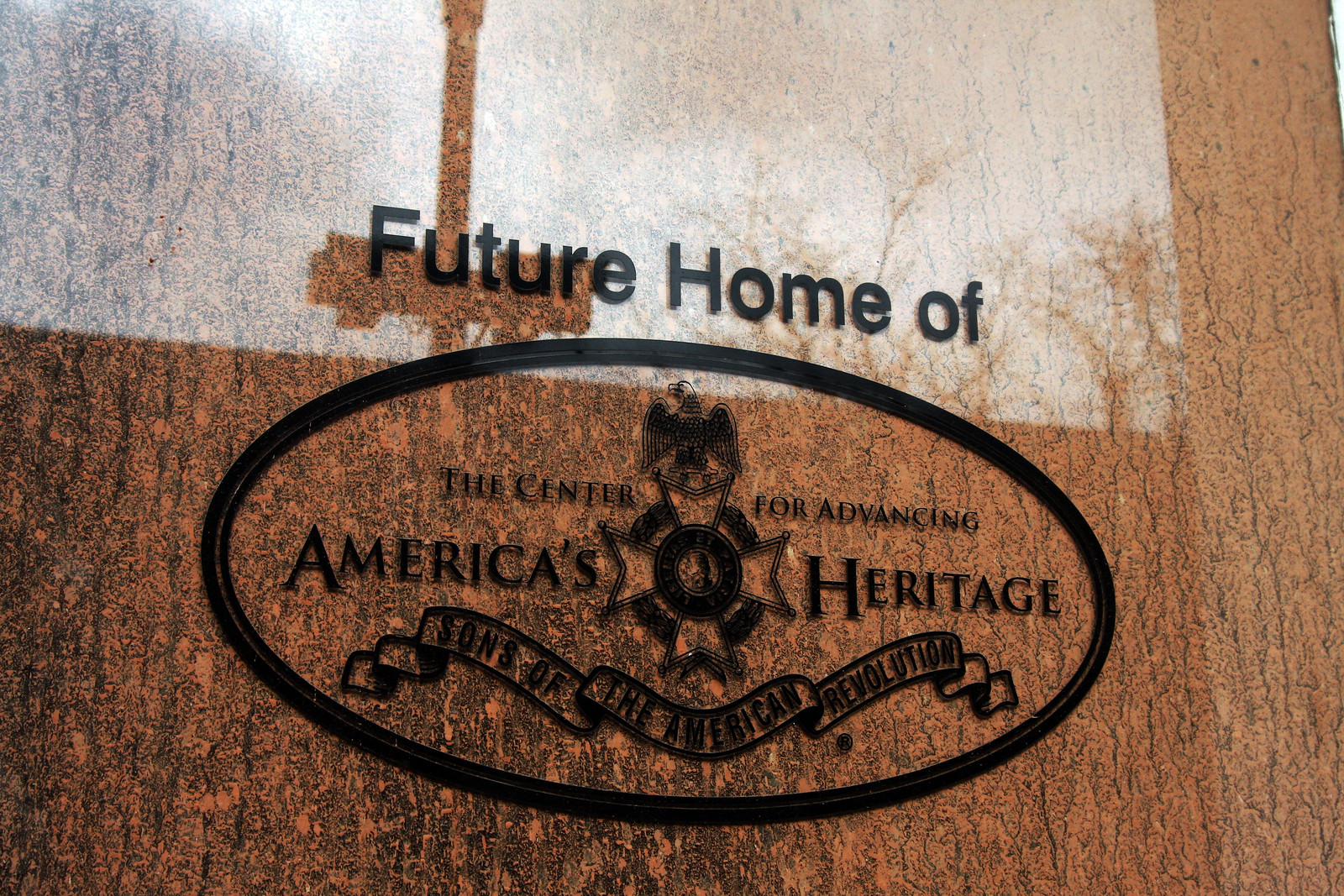This photograph captures a polished, brown-colored wall that appears to be made of marble or granite, with intricate engravings. The shiny surface of the wall reflects sunlight and possibly a pole, introducing a lighter blue hue to the top portion of the image. Central to the photograph is an inscription in black that announces the "future home of" the "Center for Advancing America's Heritage," encased within a sideways oval. Above the text sits an engraving of an eagle, and below it, a star reminiscent of an army badge or cross. Further down, a ribbon banner inscribed with "Sons of the American Revolution" completes the detailed depiction. The pattern and coloration of the wall evoke the appearance of wood, with subtle shades of brown, red, and black, emphasizing the precision and artistry of the engravings.